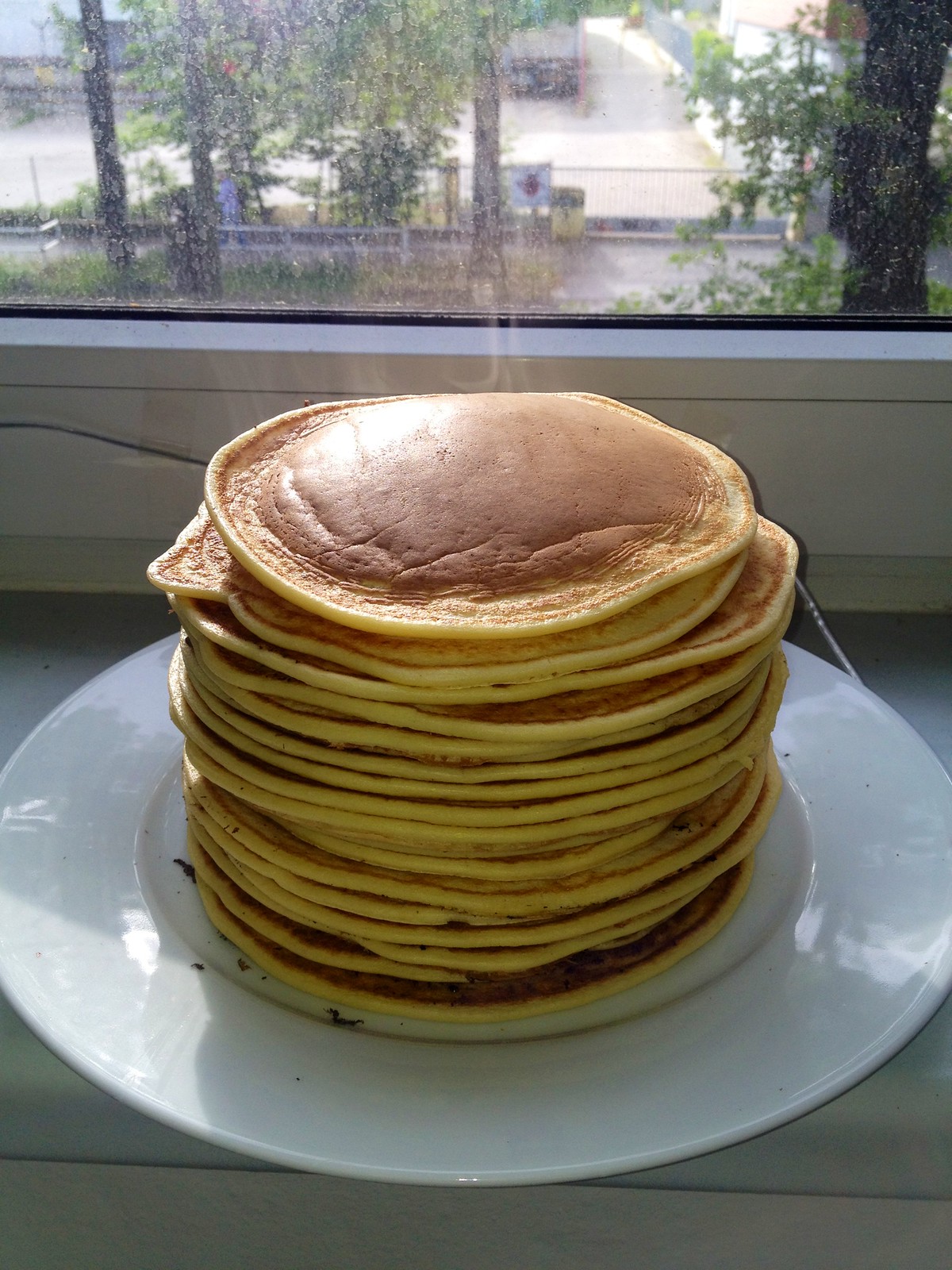A tall stack of 15 to 20 thin pancakes, perfectly browned in the middle and fading to a golden yellow around the edges, sits on a large white ceramic plate. The plate rests on a gray tabletop surface positioned on a windowsill. Through the window, adorned with a white border, sunlight streams in, illuminating the pancakes and casting a warm glow. Outside the window, the scene reveals a quiet street with a fence and gate, a few trees with green leaves, and another white building across the street. Despite the window being slightly dirty, the beauty of the bright outside world and the delicious-looking pancakes create a striking and inviting image.